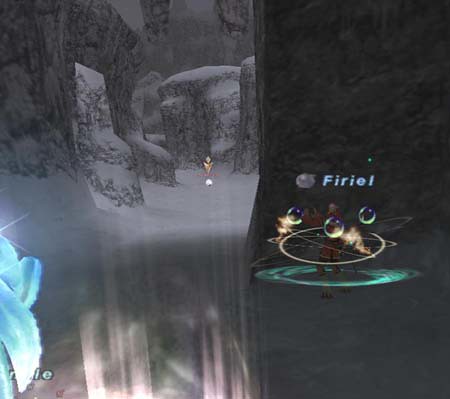The photograph appears to be a screenshot from a computer game with a slightly blurry quality, making it hard to discern the finer details. The scene has a dark and moody atmosphere, with a backdrop of dark gray clouds and possibly snow-covered terrain. In the center, there's a circle containing three characters, each with oversized bubble heads. One character stands inside the circle, another to its left, and a third figure seems to be accompanied by a bubble that isn't attached to them. Upon closer inspection, it appears that the middle character's bubble is in front of their head, and there is some smoke and a beam of blue light encircling their legs. The name "F-I-R-I-E-L" is displayed above this character.

On the left side of the image, the scene is slightly lighter in gray tones, featuring an artificial snow landscape with a large boulder in the upper left and several smaller, snow-covered boulders beneath it. The ground seems to have a shiny patch of ice near the bottom of the frame. In the lower left corner, there are blue flower petals, with an unreadable word printed on top of them that ends with the letters "-L-E."